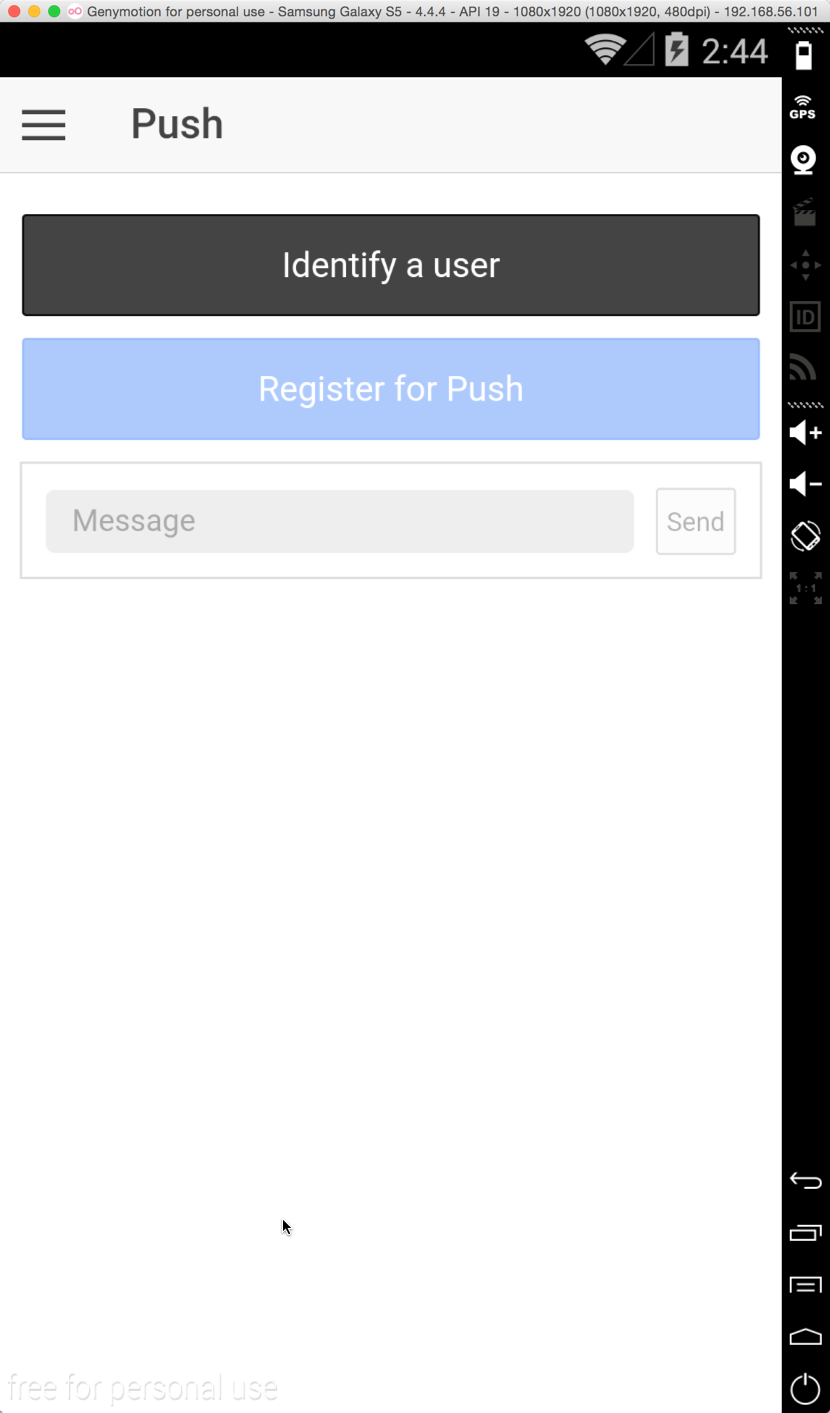The image appears to be a screenshot of a mobile emulator running on a desktop, likely Genymotion for personal use simulating a Samsung Galaxy S5 with Android 4.4.4 (API 19) and a resolution of 1080x1920 (480 DPI). 

At the top of the emulator's interface, there is a browser-like heading in light gray, featuring three circles (red, orange, and green) on the left, echoing traditional window controls. The text across the top provides technical details, including the emulator's identity and an IP address.

The emulator's layout consists of a black bar surrounding the top and right edges of the phone UI, which itself displays typical status indicators: a light gray Wi-Fi symbol, an empty signal status bar, a fully charged battery icon with a lightning bolt, and the time, 2:44.

On the right-hand vertical black bar, there's a sequence of utility icons in white: another vertical battery symbol, a GPS icon, a webcam icon, a movie icon, a navigation icon, an ID icon, and an RSS feed icon. Some of these icons appear grayed out. Additional white icons include a volume increase (+) symbol, a volume decrease (-) symbol, and a phone rotation icon.

The main content area of the phone UI shows a light gray bar labeled "push" with a hamburger menu icon to its left. Below this bar, there are three sections: 
1. A black rectangular button with rounded corners labeled "Identify User."
2. A light blue button labeled "Register for Push."
3. An outlined text field labeled "Message" with a "Send" button to its right.

At the bottom left corner is a watermark indicating "free for personal use," while a black cursor is visible near the bottom of the image, further suggesting this is a screenshot taken on a desktop environment.